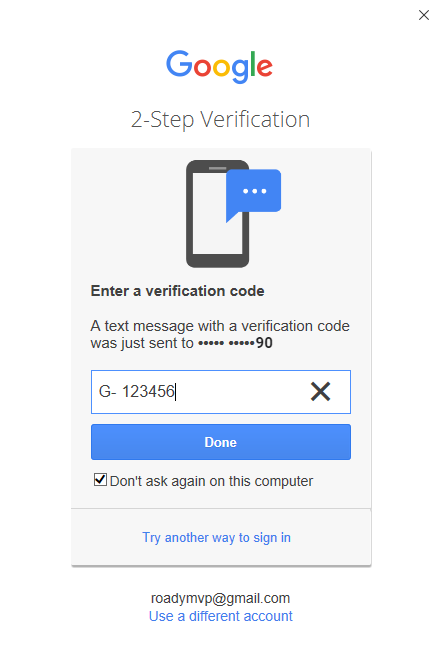The image depicts a screenshot of a pop-up menu on a mobile phone with a white background. In the upper right corner, there is a black "X" icon for closing the pop-up menu. At the top center, the Google icon is prominently displayed, featuring the word "Google" in its characteristic multi-colored font. Below this, in black text, the heading "2-step verification" is indicated.

Underneath the heading, a gray vertical rectangle encompasses the main content. At the top of this rectangle is an illustration of a smartphone or tablet with black bezels and a white screen. Emanating from the screen is a blue chat bubble containing three white dots, symbolizing an incoming message.

Further down, in black font, the text reads: "Enter a verification code." This is followed by a message explaining that "A text message with a verification code was just sent to **********90." Directly below this statement, a white input field is presented, where the user has already entered the verification code "G-123456," with the cursor blinking right after the number 6. Adjacent to this input field, on the right, there is a large "X" icon for clearing the input.

At the bottom of the pop-up menu, a blue button with the word "Done" in white text is prominently displayed, inviting the user to complete the verification process.